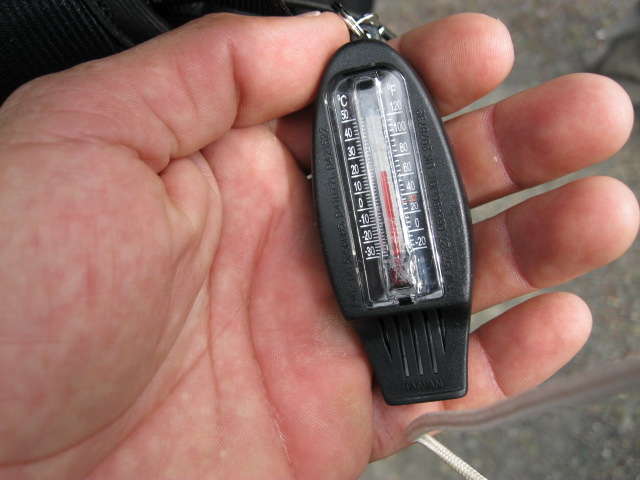In this detailed close-up photograph, the viewer's attention is drawn to the open palm of a person's hand, showcasing every finger and distinct creases along the skin's surface. In the space between the thumb and forefinger, the individual is holding a black, temperature-measuring device approximately five inches in length. The device features a silver keyring at its top, suggesting portability.

On the left side of the device, the letter "C" is visible at the top, followed by a descending series of numbers: 50, 40, 30, 20, 10, 0, -10, -20, and -30, representing temperatures in Celsius. The right side mirrors this with the letter "F" above a corresponding series for Fahrenheit: 120, 100, 80, 60, 40, 20, 0, and -20. Centrally positioned on the device, a thin, red indicator line hovers near 60 degrees Fahrenheit, aligning closely to 20 degrees Celsius.

Extending about two inches below the thermometer scale is a black tab, also grasped within the person's hand. Noteworthy is a slender white string visible in the photo's lower right corner, suggesting the thermometer might be attached or related to something else.

The image background reveals a smooth, gray surface, possibly a floor or countertop, providing a neutral contrast to the hand and the object. The close-up clarity allows for visibility of tiny red dots on the person's skin, underscoring the intimate and tactile nature of this photograph.